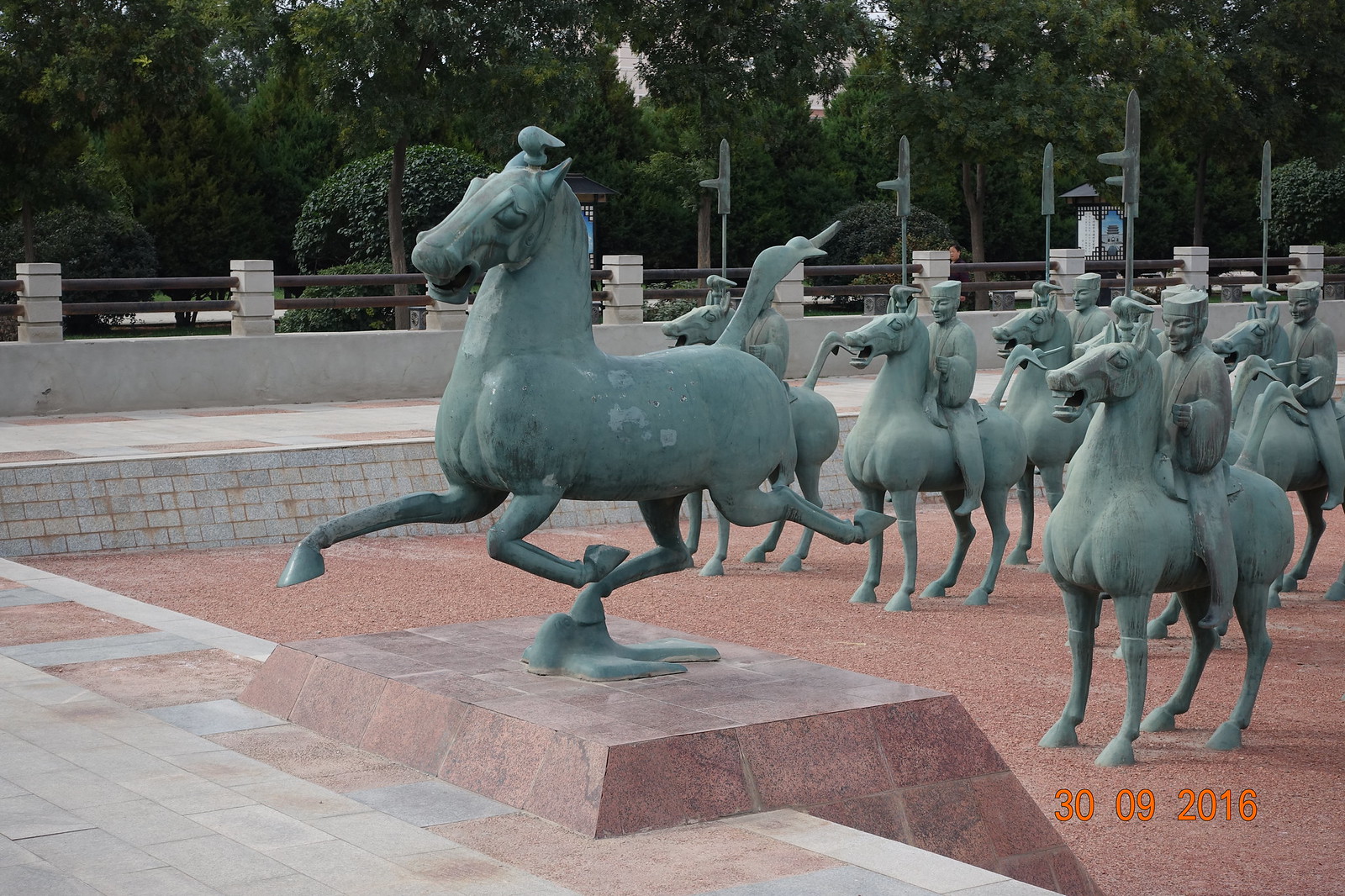In this detailed outdoor photograph dated September 30, 2016, we see a row of statues set against a backdrop of lush green trees and neatly trimmed bushes. The statues are situated in a park-like setting with a pink-colored, marble-tiled platform. The forefront of the image features a prominent galloping bronze horse with a turquoise patina, mounted on a small pedestal on a coral marble base positioned near marble stairs. This lead horse is depicted without a rider and has three of its legs mid-air. Behind it, several statues of other horses stand still with all four legs grounded. Each of these horses carries a rider, sculpted to resemble Asian men wearing square hats. The platform beneath the horses transitions to a reddish, clay-colored pavement, enclosed by a fence with white concrete posts connected by black metal rods. The entire scene captures an arrangement of horse statues with riders in a meticulously landscaped park, captured in a crisp digital photograph.